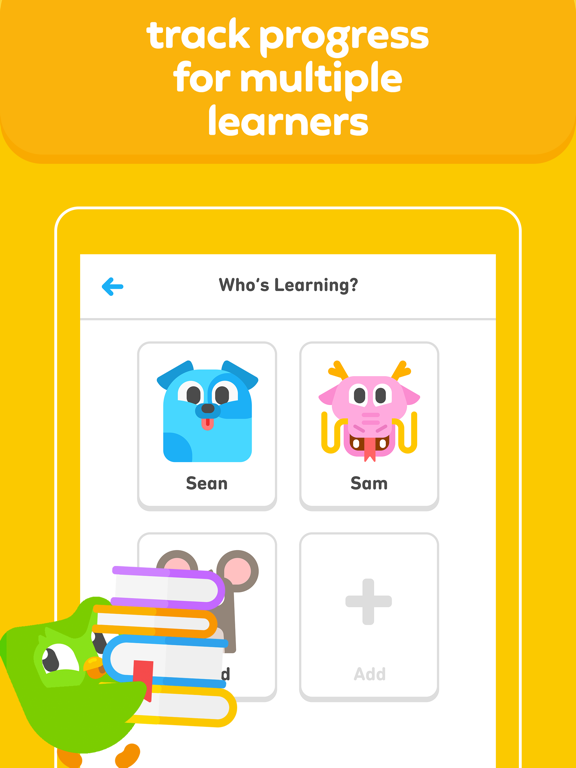"Illustration from an online app with a vibrant yellow background, featuring various colorful elements designed to promote learning progress tracking for multiple users. At the top, in bold white text, the phrase 'Track Progress for Multiple Learners' is prominently displayed. Below this headline, a white triangle and a white rectangular form are positioned, with the latter containing the text 'Who's Learning' accompanied by a blue arrow pointing to the left.

The image also includes playful cartoon characters: a blue dog labeled 'Sean,' and to its right, a pink creature with yellow horns named 'Sam.' Adding to the whimsical scene, a charming green bird with a yellow beak is seen at the lower left, carrying a stack of four books, symbolizing educational growth and curiosity."